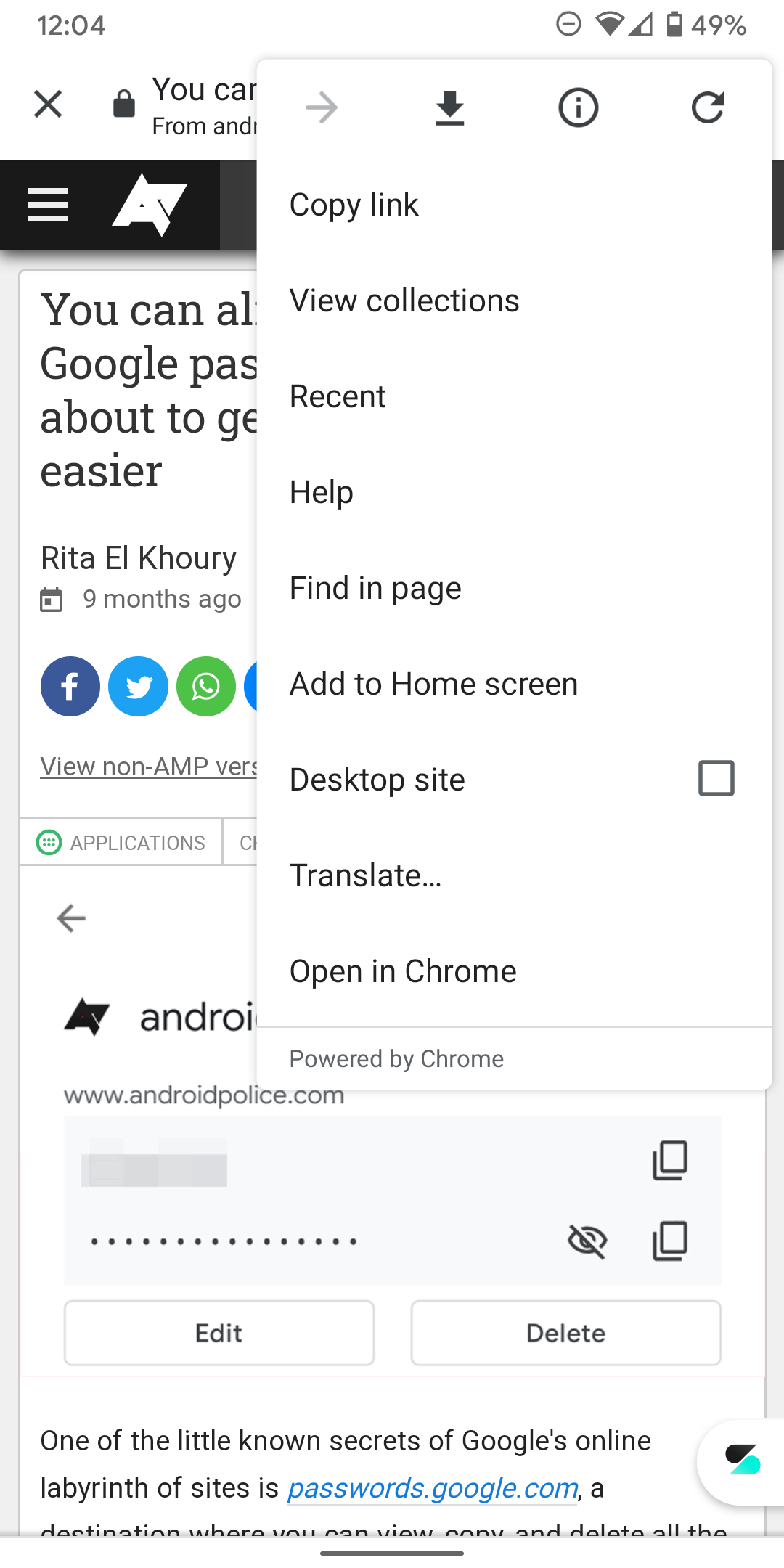The image is a screenshot from an Android phone, showcasing a webpage. At the top right corner, the phone's status bar indicates a battery level of 49%, depicted by a vertical battery icon. Adjacent to the battery icon is a signal strength indicator showing one or two bars, and a nearly full Wi-Fi signal icon, probably indicating three or four bars. The top left of the screen displays the current time of 12:04.

Dominating the middle right section is a vertical rectangular pop-up overlay with four icons at the top: a right-pointing arrow, a download icon, an information icon (a lowercase "i" inside a circle), and a refresh icon represented by an arrow in a circle. The left side of this pop-up lists several options: "Copy link," "View collections," "Recent," "Help," "Find in page," "Add to home," and "Desktop site." The screenshot captures a snapshot of the phone interface with a focus on the webpage and the browser's menu options.